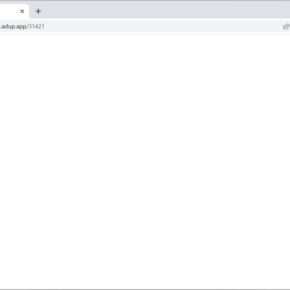This image features a minimalistic, predominantly white screenshot that seems to be from an internet search engine page. The central focal point is a very small portion of a light gray search bar, partially visible at the top of the screen. The screenshot is noticeably cropped, cutting off most of the interface and providing a fragmentary glimpse into the webpage. Above the search bar, a slightly darker gray taskbar is visible, indicating the presence of an open tab, although the text within this portion is too small and blurry to decipher. The absence of any objects, text, or distinctive layout renders this image void of any useful or discernible information. The uniform white background and the lack of any significant details contribute to an overall impression of emptiness and minimal content.